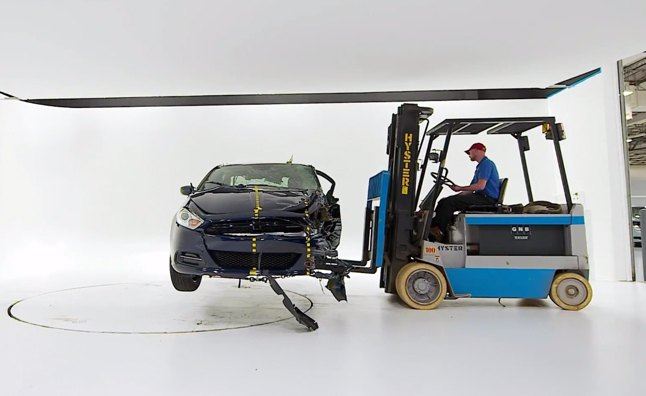The photograph depicts a man in a blue, black, and light gray Hyster forklift, lifting a heavily damaged black sedan. The man, dressed in a blue short-sleeved shirt, black pants, and a red baseball cap, operates the forklift inside a stark white room with white floors, walls, and ceiling. The sedan, which is facing the viewer, has been wrecked on its right side, leaving the left side mostly intact. Yellow dots are painted down the center of the car, which is being raised above a large black circle painted on the floor, likely indicating a safety testing area. The remains of the front bumper and fender are partially hanging off, with some pieces touching the ground.